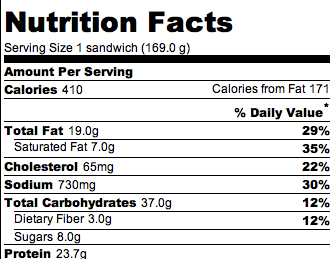The image displays a nutrition label against a stark white background with black text. Titled prominently in large font, "Nutrition Facts," it outlines detailed nutritional information for a serving size of one sandwich, which weighs 169 grams. The label records that the sandwich contains 410 calories, with 171 of those calories coming from fat. The total fat content is 19 grams, making up 29% of the daily value, and includes 7 grams of saturated fat, which is 35% of the daily value. Cholesterol is listed at 65 milligrams (22%), while sodium content is notably high at 730 milligrams, equaling 30% of the daily value. The sandwich also contains 37 grams of total carbohydrates (12%), which includes 3 grams of dietary fiber (12%) and 8 grams of sugar. Protein content is 23.7 grams. There is no additional information or comparative daily value chart at the bottom of the label. The overall design is highly contrasting with its black and white color scheme, ensuring the information is clear and easy to read.